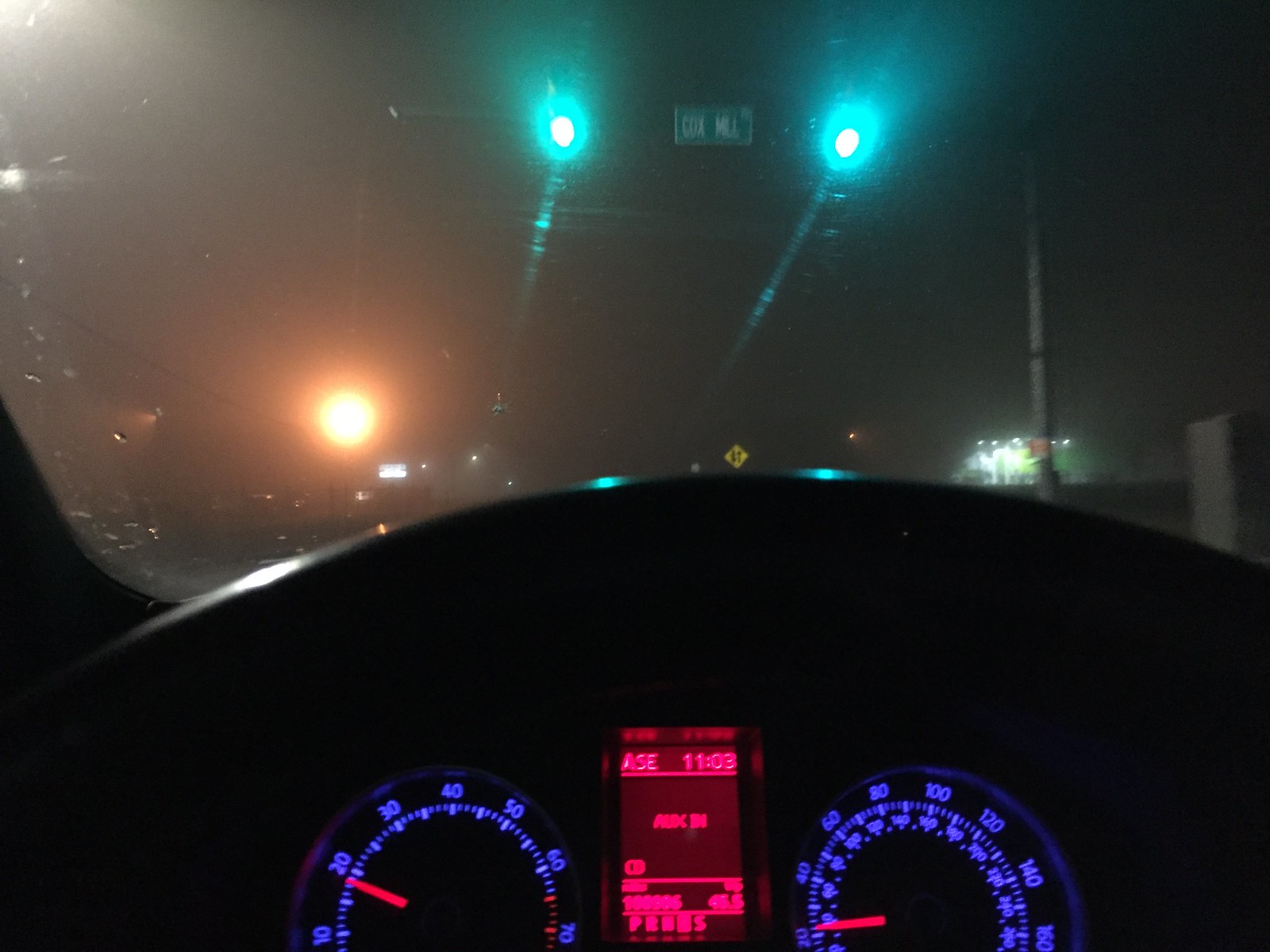This vibrant nighttime photograph captures the driver's side perspective of a vehicle's interior. Dominating the lower third of the image, the dashboard is illuminated by a soft, ambient light. The analog speedometer to the left is distinct with its bright purplish-blue numbers and striking red dial indicator. Centrally positioned are additional illuminated instrument readings, though their specifics are unreadable. To the right, another dial is visible. Through the windshield, the scene outside reveals a nighttime intersection marked by green traffic lights. Off to the left, a streetlamp casts a subtle glow, enhancing the nocturnal ambiance.